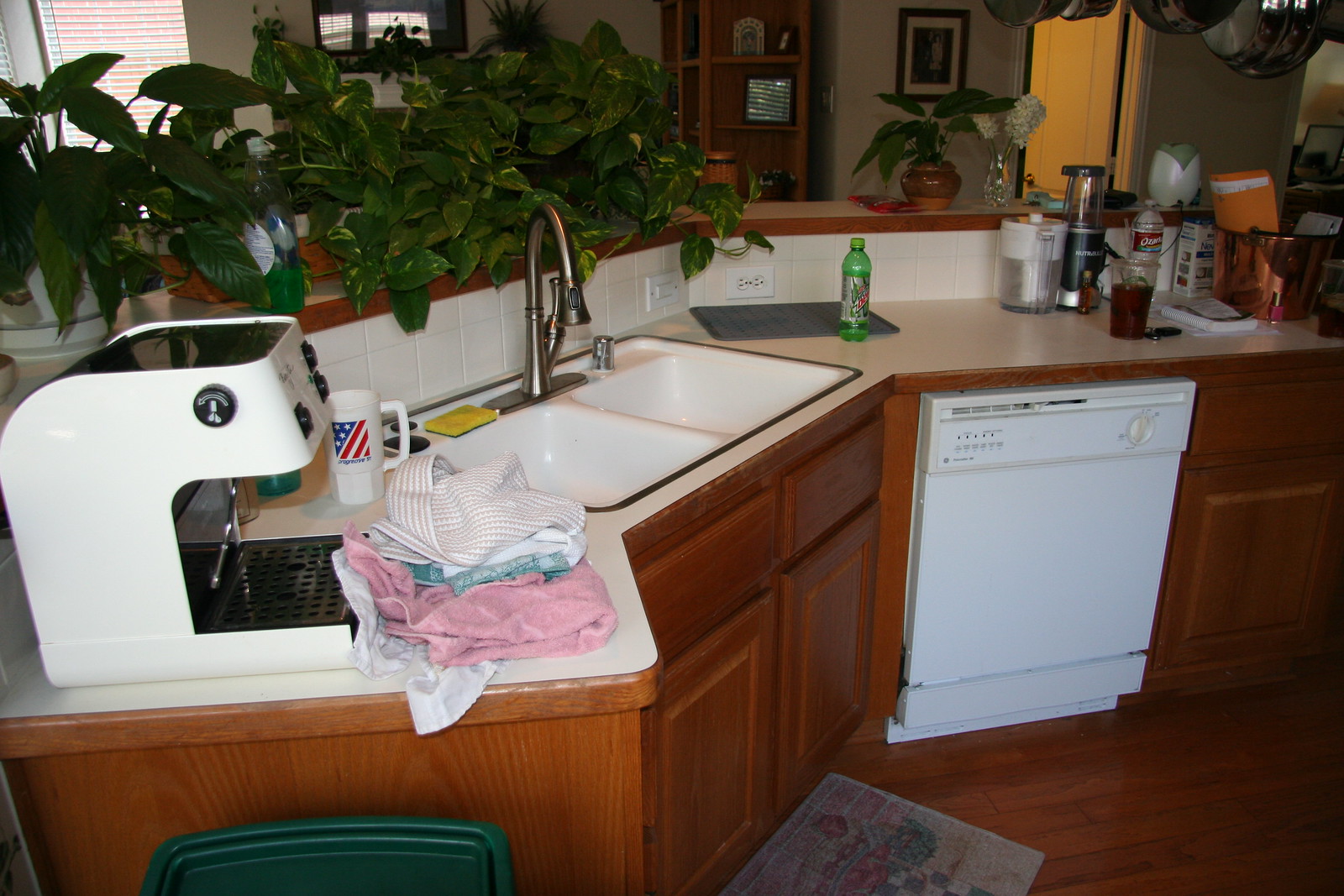The image captures a bustling kitchen scene centered around a spacious island-style counter in a cozy home. On the counter, draped with a few cloth items, sits a white sink with a gleaming metal faucet. To the left, at the bottom of the photo, a white coffee machine with black buttons stands alongside neatly folded cloths. Next to the sink, a white mug adorned with an American flag pattern sits prominently, while a yellow sponge with a green underside rests on the sink's edge. Moving right across the counter, a green and gray Mountain Dew bottle catches the eye.

Adjacent to the counter, a white dishwasher is positioned under brown cabinets, and atop the counter above the dishwasher lie various items including a pitcher, some supplies, a glass filled with a beverage, and an empty soda bottle. In the background, an open door is visible in the upper right corner, next to which a picture frame with a painting hangs. Below the painting sits a vase filled with plants, adding a touch of greenery to the space. A shelf with assorted decorations is also visible, along with numerous plants perched above the counter. A window in the background lets in natural light, illuminating the wooden floor. On the bottom left, a green trash bin is noticeable, while a brown floor mat spreads out in front of the sink, enhancing the homely atmosphere.